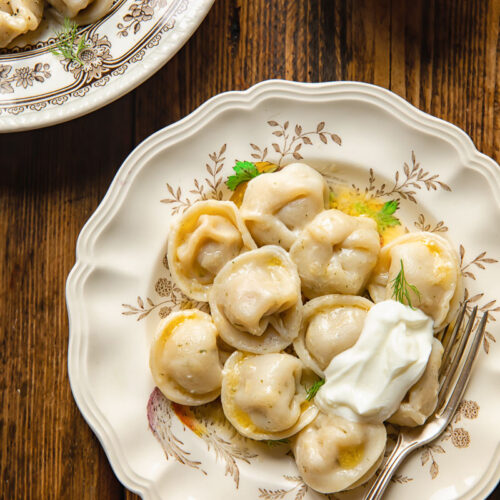This photorealistic image captures an overhead view of a beautifully set wooden table featuring two plates of food. The main focus is on a decorative plate with intricate scalloped edges and floral or plant designs. This plate contains a serving of golden, dumpling-like gnocchi, topped with a dollop of white cream, possibly sour cream or yogurt. A silver fork rests elegantly on the plate, adding to the refined presentation. The table itself is a light wood grain, enhancing the rustic yet sophisticated atmosphere. In the upper left corner of the image, another plate peeks into view, bearing a different floral and leaf pattern, though its contents remain unseen.